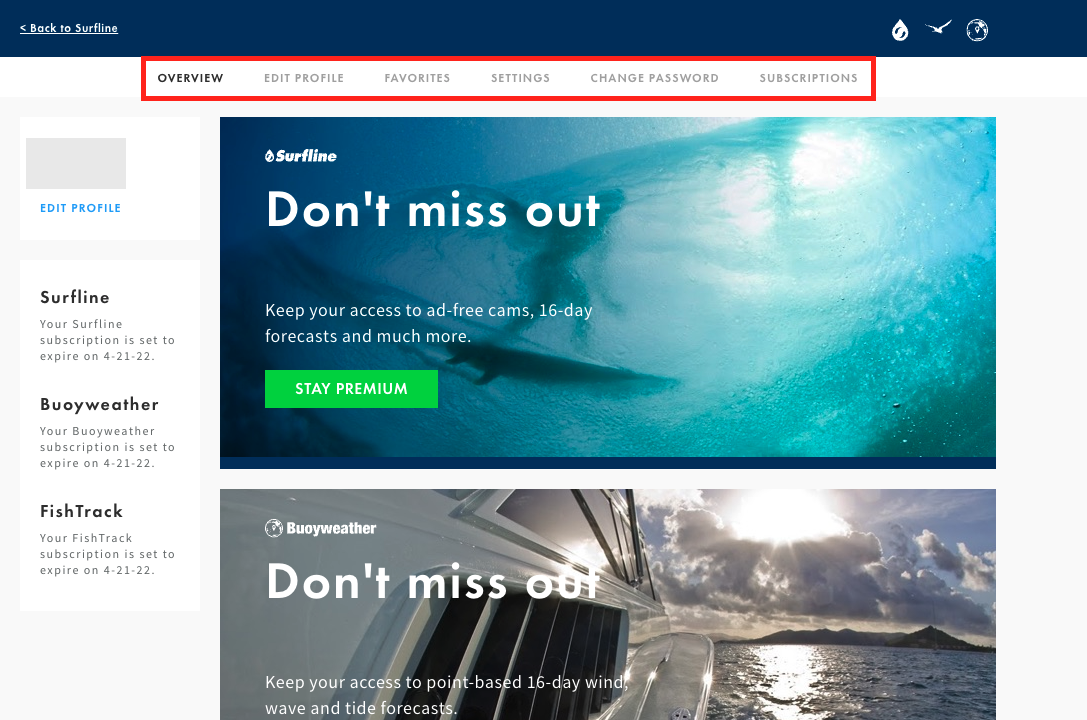**Caption:**

The image is a screenshot from a website, specifically from a page under the Surfline domain. At the top of the screenshot is a dark blue rectangular navigation bar with a left-pointing arrow and a hyperlink labeled "Back to Surfline," indicating this page is part of a larger navigational flow. In the top right corner of the bar, three small icons are visible: a water droplet, a flying bird, and a globe with a location marker in the center, likely representing various site functionalities or sections.

Highlighted with a red rectangle, the main navigation menu runs horizontally across the top of the page and includes six options: Overview, Edit Profile, Favorites, Settings, Change Password, and Subscription. Along the left-hand side of the webpage, a vertical menu continues the theme of profile management, situated against a white background.

Dominating the main body of the webpage are two large images related to surfing. The first image shows an underwater view of the sea, overlaid with text encouraging users to maintain their premium access for benefits like ad-free live cams and 16-day weather forecasts. Below it, a green button prompts, "Stay Premium." The second image features a side view of a boat on the ocean, with overlaid text emphasizing the continued access to detailed 16-day wind, wave, and tide forecasts. Both images and their accompanying texts underline the site's focus on providing comprehensive resources for surfing enthusiasts.